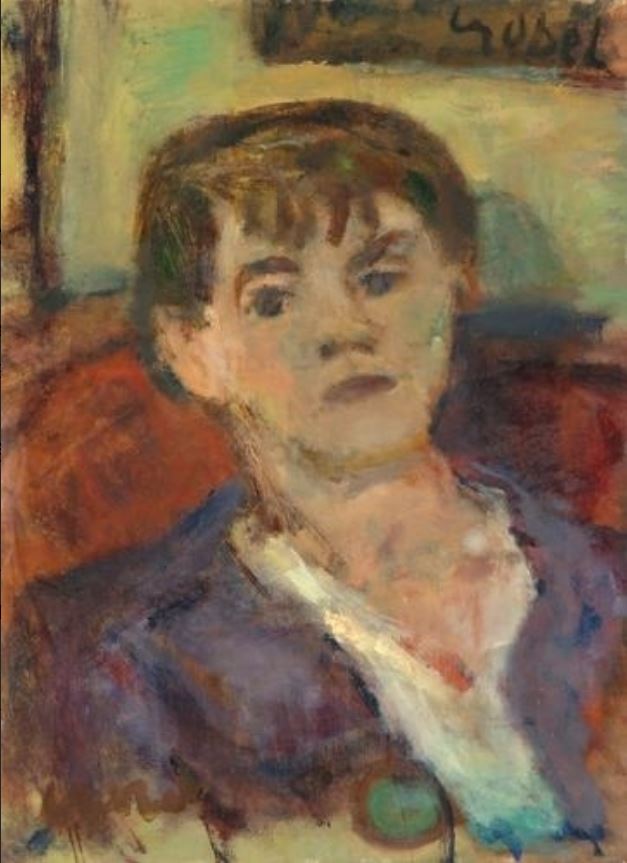This painting, titled "Noe Portrait" by artist Viraj Judit, exemplifies an Impressionistic style. It captures a boy with short, dark reddish-brown hair adorned with bangs, and blue eyes, who is slightly smiling as he looks toward the viewer. The child, centrally positioned in the composition, appears to be reclining on a red couch. His attire includes a white shirt, open at the chest, beneath a blue overcoat. A notable detail is a gray circular object with a greenish hue, located at the bottom center of his jacket. The background features a beige wall with a window and a brown painting above the couch. The colors used in the painting are varied, including black, brown, green, tan, orange, red, turquoise, pink, and purple, contributing to the rich, splotchy texture characteristic of the Impressionist technique. In the upper right corner, the artist's signature is visible. The portrait, oriented vertically, occupies the majority of the frame, emphasizing the boy as the focal point in an indoor setting.